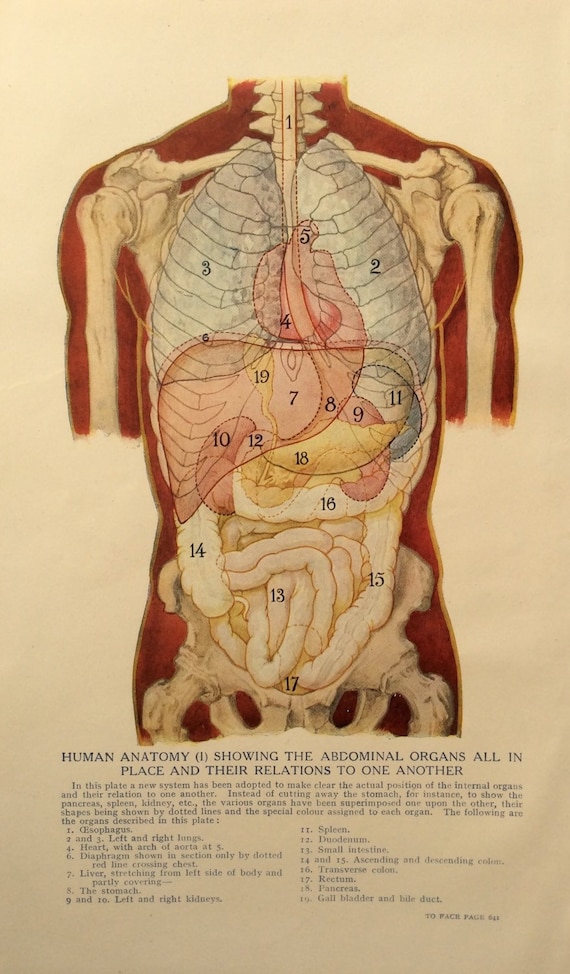This image is a detailed vintage color illustration of the human torso from the neck to mid-hips, extracted from an old anatomy textbook or publication. Its age is evident from the beige discoloration of the page and the period-specific font styles. The portrait-oriented image focuses on the internal anatomy of a human male, depicting the organs in a frontal view, all meticulously numbered from 1 to 19. The illustration, rendered in color, vividly displays various organs: the blue-tinted lungs at the top, the pink stomach, the yellow liver, and variously shaded intestines. The underlying bone structure is visible but not the focus. 

Beneath the illustration, a headline reads "Human Anatomy (1)," specifically indicating the arrangement and relationships of the abdominal organs. There is a numerical key coding system, with each number corresponding to a black text explanation of the organ names, detailed in a slightly hard-to-read descriptive text at the bottom. The background mimics aged parchment, adding to the vintage aesthetic of the publication. The area around the depicted structures is colored in a dark brick red, enhancing the contrast and visibility of the organs.